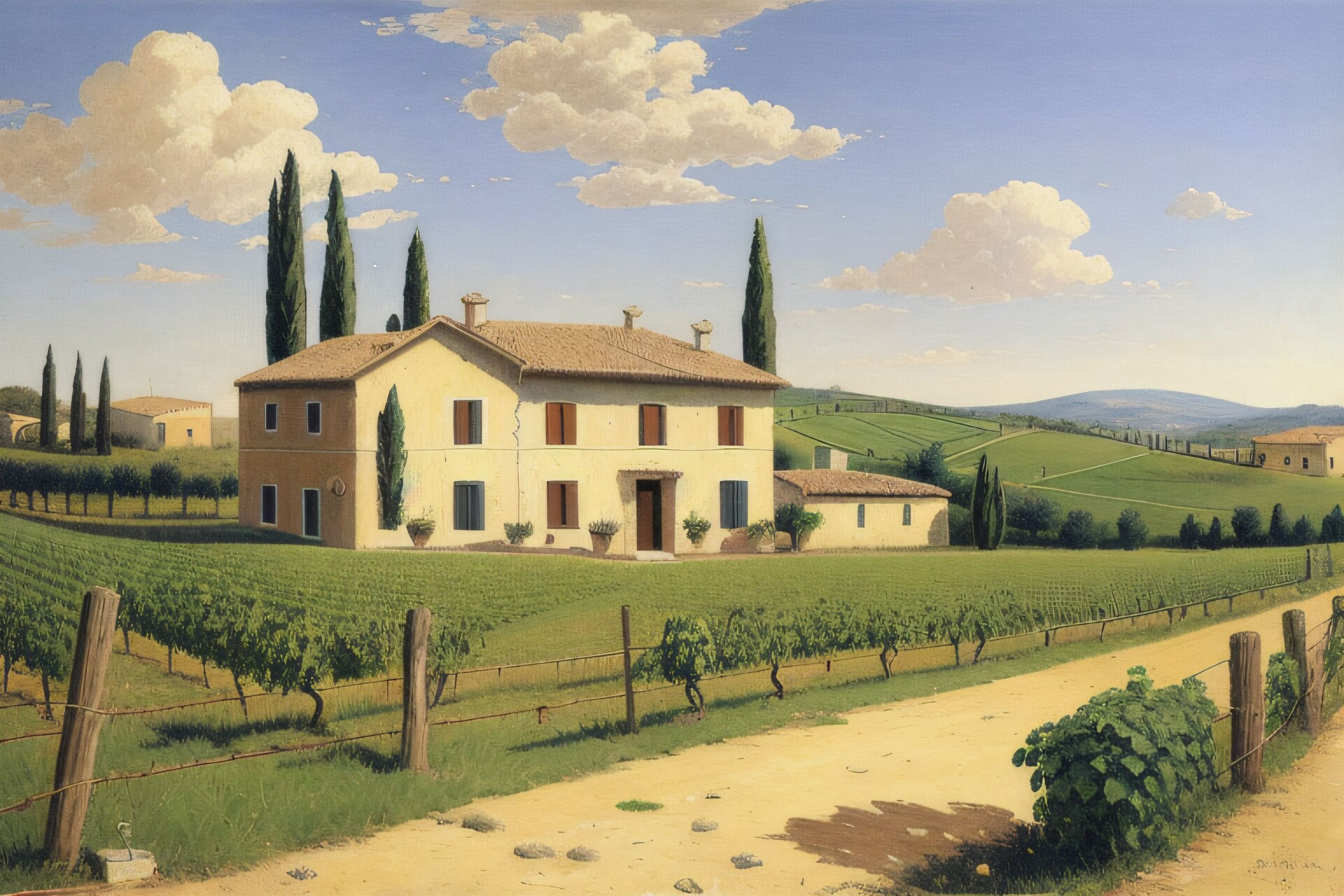This image appears to be an oil painting, potentially created by AI, depicting a rustic two-story villa, possibly situated in the European countryside such as Italy or Spain. The villa features a front and side vineyard, with greenery that becomes spotty beyond the first rows. The house has a front brown door and is surrounded by shrubs and flowering plants growing along wooden pillars. The scene includes a barbed wire fence running parallel to a dirt road in front of the villa, which curves off to the right. Behind the house, there are a few tall trees, and in the far distance, a mountain or hill range can be seen under a clear blue sky with a few scattered clouds. Additional farm buildings are present in the background amidst rolling hills and open plots of grass. Notably, a hovering bush or tree near the house and inconsistencies in the fence's appearance hint at its AI-generated nature.